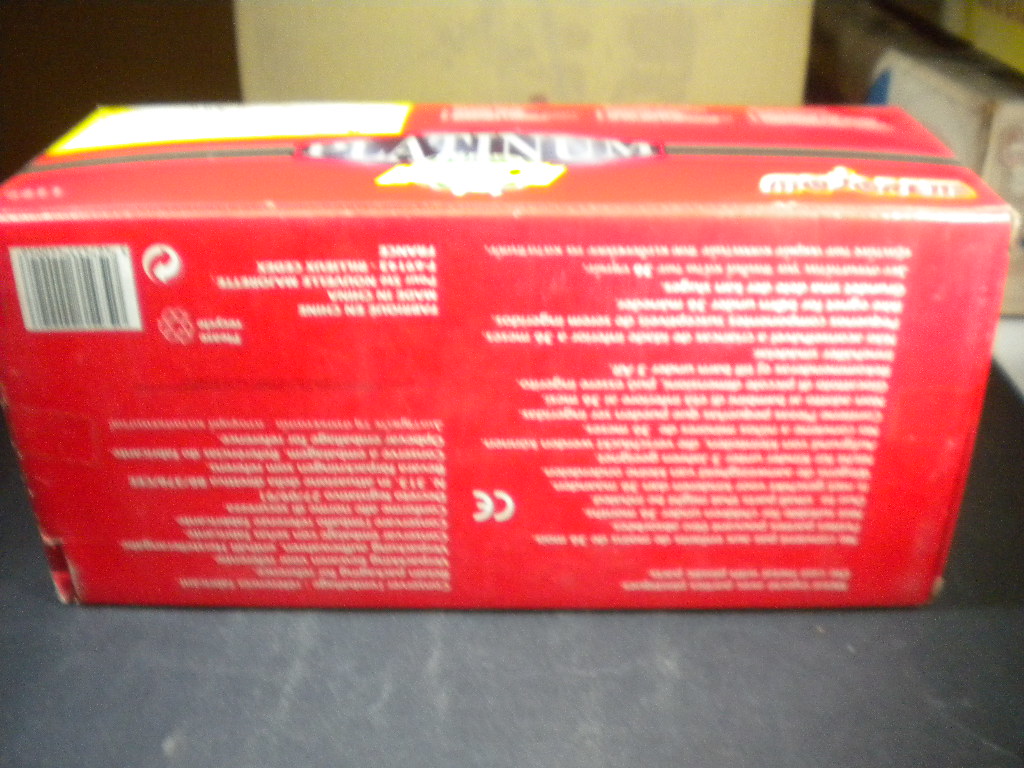The image features a vibrant red box positioned upside down on a dark gray surface, suggesting a setting within a warehouse or storage area. In the background, various other items are visibly stored, including a distinct gold-colored box. The red box, adorned with white lettering, prominently advertises "Platinum," though the text is inverted from the viewer’s perspective. The box is designed to open from the top, where a long slot is clearly visible. Atop the red box rests a white box trimmed in yellow, accompanied by a noticeable UPC symbol.